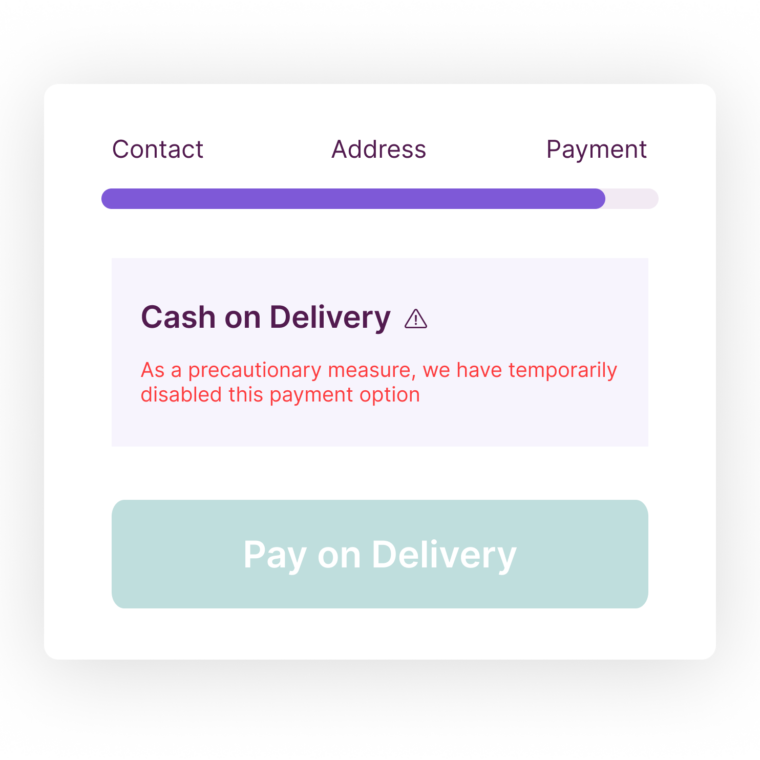The image features a gray background with a central white square displaying various payment-related information. Within the square, there are several elements:

1. A purple bar titled "Contact Address Payment" that nearly touches the end, indicating 80% completion.
2. Below this bar is a gray rectangle with text reading "Cash on Delivery."
3. To the side, there is a red triangle with an exclamation mark, accompanied by the message "As a precautionary measure, we have temporarily disabled this payment option."
4. Beneath the red triangle, a blue rectangle contains the words "Pay on Delivery" in white text.

The elements are arranged to clearly indicate the payment options and current limitations on the "Cash on Delivery" service.